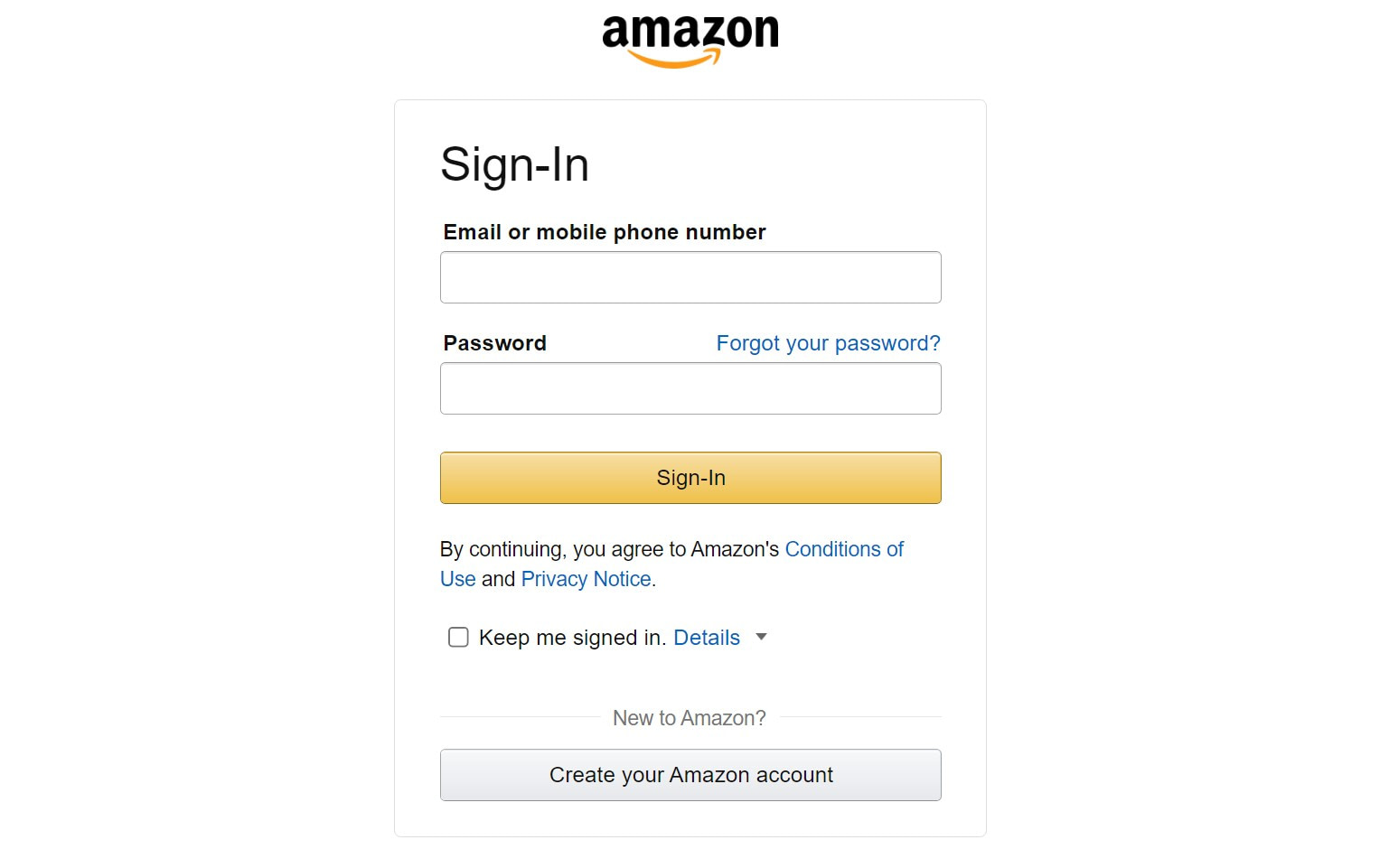An image of the Amazon sign-in page is depicted with a clean, white background. Centrally positioned at the top, the bold, black "Amazon" logo is prominently displayed, extending from "A" to "Z" with the iconic gold arrow swooping down and then up to the right. Below the logo, a thin black border frames the sign-in section, running along the top, sides, and bottom.

In the top left corner of this bordered area, the word "Sign-In" appears in large, bold black letters. Directly beneath, it reads "Email or mobile phone number" in smaller, but equally bold, black text. A white rectangular input field is provided for users to enter their email or phone number.

Further down, the word "Password" is similarly bolded in black, with a blue "Forgot your password?" link to its right. A second white input field is positioned below this for users to enter their password. 

An orange button, centered, bears the word "Sign-In" in black, inviting users to continue. Below this button, a statement in black reads, "By continuing, you agree to Amazon's," with "Conditions of Use" and "Privacy Notice" hyperlinked in blue.

There is a checkbox with a white background and black border labeled "Keep me signed in." To its right, the word "Details" is printed in blue with a small dropdown arrow.

Towards the bottom center in light gray text is the prompt "New to Amazon?" Directly below this, a wide gray button spans the page, containing the text "Create your Amazon account" in black.